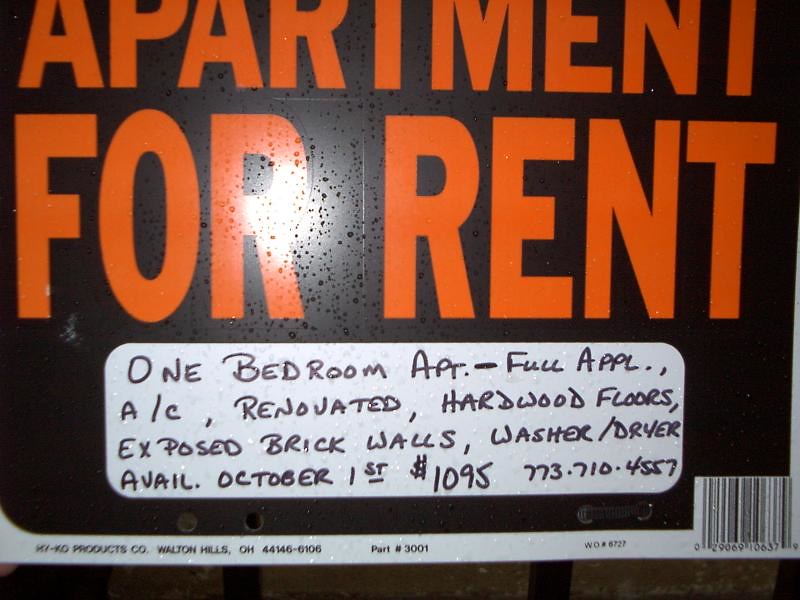In this advertisement for an apartment for rent, bold orange letters on a black background announce "Apartment for Rent," though the top part of the word "apartment" is cut off. The sign, which appears to be wet with water droplets and photographed at night using a camera flash, features detailed information handwritten in a white space below the main heading. The apartment is described as a one-bedroom unit with full appliances, air conditioning, recent renovations, hardwood floors, exposed brick walls, and a washer and dryer. It becomes available on October 1st, for a monthly rent of $1,095. For inquiries, the contact number provided is 773-710-4557. The bottom of the sign contains a partial barcode and some unrelated text that includes "Walton Hills, OH 44146-6610" and the partially obscured phrase "tag 3001" amidst other unreadable elements.